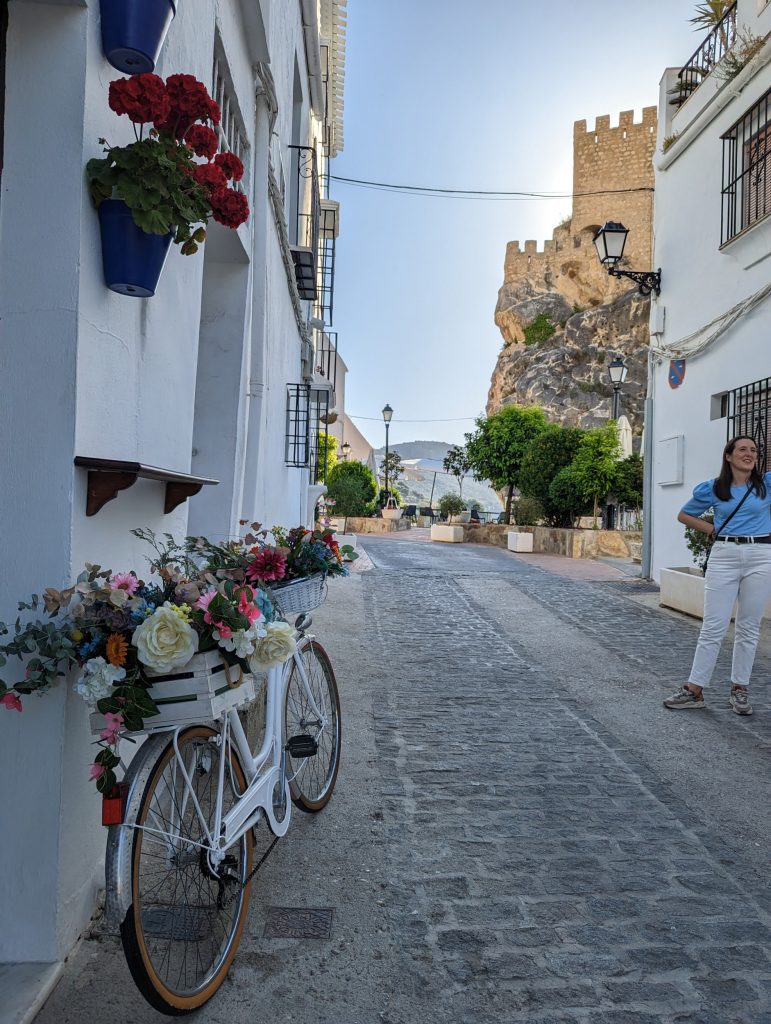A picturesque street scene likely set in Europe, possibly Spain, features a quaint cobblestone alley with tall, charming buildings on either side. The foreground displays a vintage single-seat white bicycle with tan and black tires, leaning against a building on the left. Its baskets overflow with a vibrant array of flowers, adding a burst of color to the setting. Adjacent to the bicycle, a hanging pot of red flowers decorates the wall. 

To the right, a young woman with medium-length hair and a pleasant smile stands near the entrance of a building. Dressed in a blue peasant-like top, white pants, a black belt, and sneakers, she appears to be engaged in a conversation, enhancing the candid travel moment. Above her, a streetlamp affixed to the building casts a gentle light.

In the distance, beyond the rows of classic buildings adorned with intricate balconies and floral pots, a majestic stone fortress or castle, likely made of sandstone or yellow brick, stands against the horizon. The serene mountain range further adds depth and enchantment to the scene, making this a captivating snapshot of everyday beauty and architectural charm.